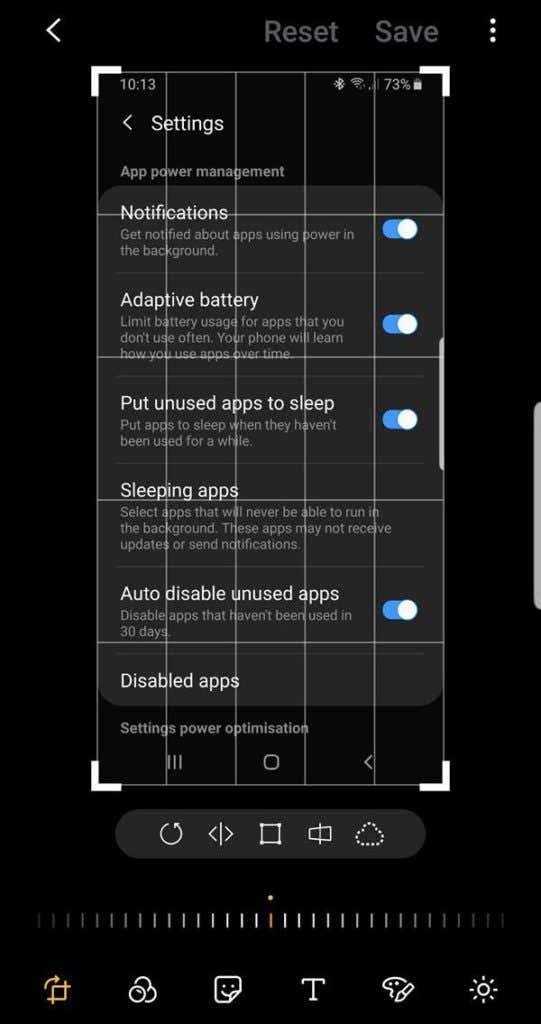The image depicts a smartphone settings interface overlaid with a white grid on a black background. In the upper left corner, a large white arrow pointing left is prominently visible. Adjacent to this, "1013" is displayed, indicating the time. To the right, app control options titled "Reset" and "Save" are visible in gray text, and further right, three white dots are arranged vertically, signifying a menu or more options.

The phone screen shows several status icons: Bluetooth, Wi-Fi, and cell signal bars, along with a battery indicator showing 73% remaining. The screen is currently on the "Settings" page, which is indicated by a left arrow next to the word "Settings" at the top. Below this, the heading "App Power Management" is displayed.

Underneath the heading, various options related to power management are listed:
1. "Notifications: Get notified about apps using power in the background." This option is toggled on, highlighted in blue.
2. "Adaptive Battery: Limit battery usage for apps that you don't use often. Your phone will learn how you use apps over time." This option is also toggled on.
3. "Put unused apps to sleep: Put apps to sleep when they haven't been used for a while." This option is toggled on.
4. "Sleeping apps: Select apps that will never be able to run in the background. These apps may not receive updates or send notifications."
5. "Auto disable unused apps: Disable apps that haven't been used in 30 days." This option is toggled on.

At the bottom of the list, there is an option labeled "Disabled apps," but the text below it is not fully visible in the image. The white grid overlay, with bolded corners and thin lines forming a grid pattern, adds an additional layer of visual structure to the image.